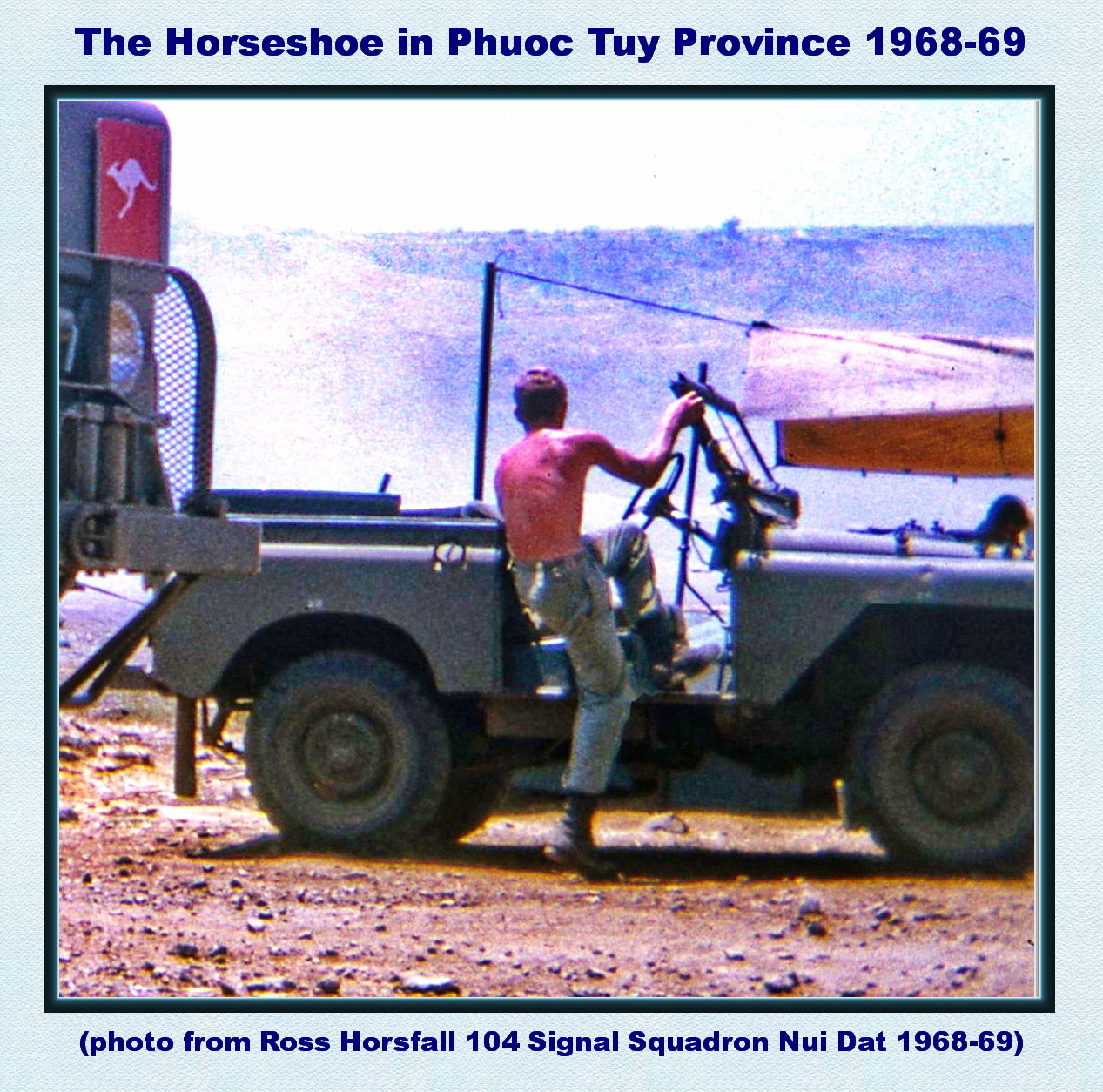This historical photograph, framed with a light blue border, captures a young soldier facing away from the camera, climbing into the passenger side of a topless, army green Humvee. The soldier, topless and wearing army green pants and boots, is the focal point of the image, set against a backdrop of dirt, rubble, and a distant, rolling hill. The scene is shrouded in a smoky haze, indicative of the rugged, dusty terrain. To the left in the foreground, you can see the front grille of another vehicle, distinguished by a red square featuring a running kangaroo. The image is suggestive of an Australian setting. A makeshift tent, supported by a post and string, is visible near the Humvee. The caption above the photograph reads: "The Horseshoe in Phuoc Tuy Province, 1968-69," while below, it notes: "(Photo from Ross Horsefall, 104 Signal Squadron, Nui Dat, 1968-69)."